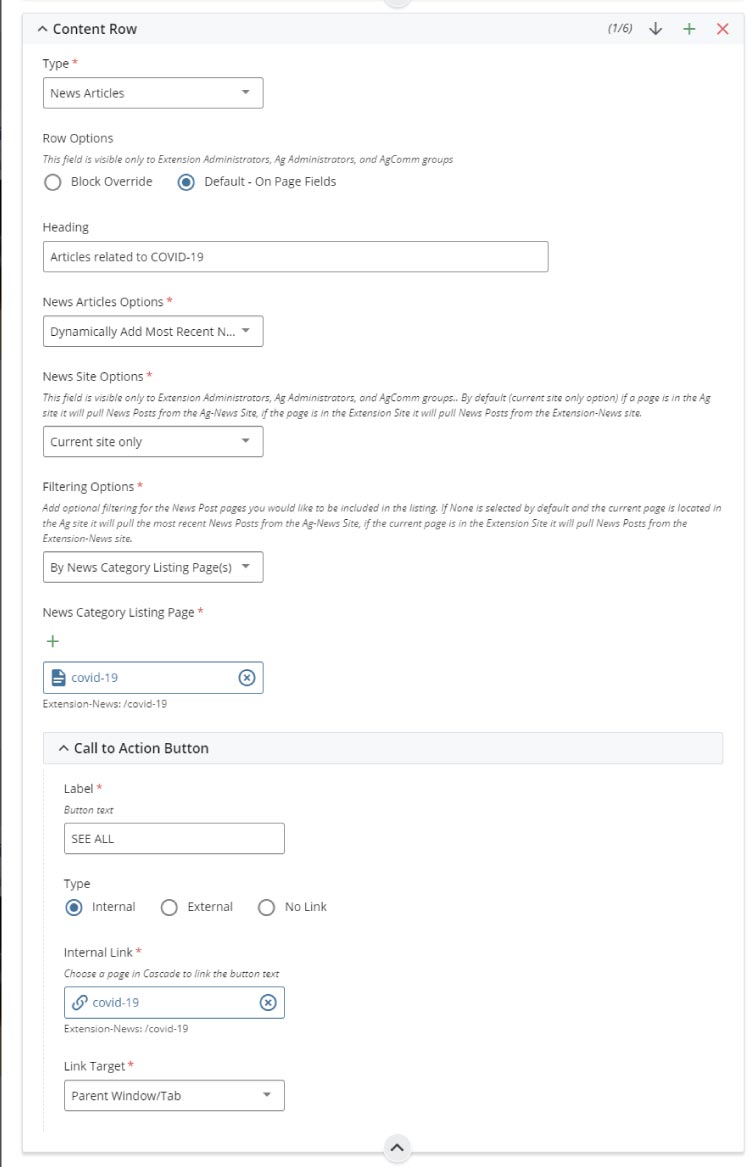In the image, there is a detailed webpage interface featuring multiple settings and options. The page has a clean, white background with black font. At the very top, there is a heading labeled "Content Row" followed by a section titled "Type" with a drop-down box set to "News Articles." 

Below this, we encounter the "Row Options" section, which includes a notification stating that this field is visible only to specific groups: Extension Administrators, AG Administrators, and AG Comm Groups. The section also contains clickable options labeled "Block," "Override," and "Default."

Further down, there is a "Heading" field with the text "Articles related to COVID-19." Beneath the heading, the "News Article Options" section features a drop-down box with the option "Dynamically Add Most Recent."

The next section is titled "News Site Options," which, similar to "Row Options," is restricted to specific user groups. It includes a drop-down box labeled "Current Site" with the option "Current Site Only."

Following this, the "Filtering Options" section appears, featuring a drop-down box labeled "By News Category Listing Pages." Within this section, another sub-section titled "News Category Listing Pages" includes a box containing the text "COVID-19."

Each element on the webpage is clearly defined and structured, indicating an interface designed for managing news content, specifically related to COVID-19.